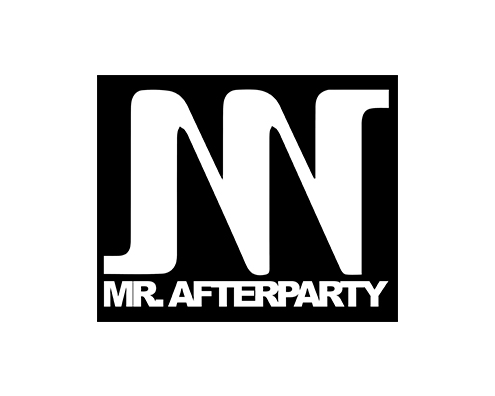The image is a black square featuring a predominantly white graphic and text. The primary graphic, occupying about 90% of the image, is a stylized, continuous zigzag pattern resembling an 'M.' This stylization includes three peaks and three dips, with a thick left side and thinner, more tapered right downward slopes, giving it a wave-like appearance. Below this intricate design, the text "Mr. Afterparty" is prominently displayed in white block letters. The "Mr." is abbreviated with a period, and "Afterparty" is presented as one word, tightly packed into the remaining 10% of the image. Both elements—graphic and text—contrast starkly against the black background, making the design and lettering stand out vividly.